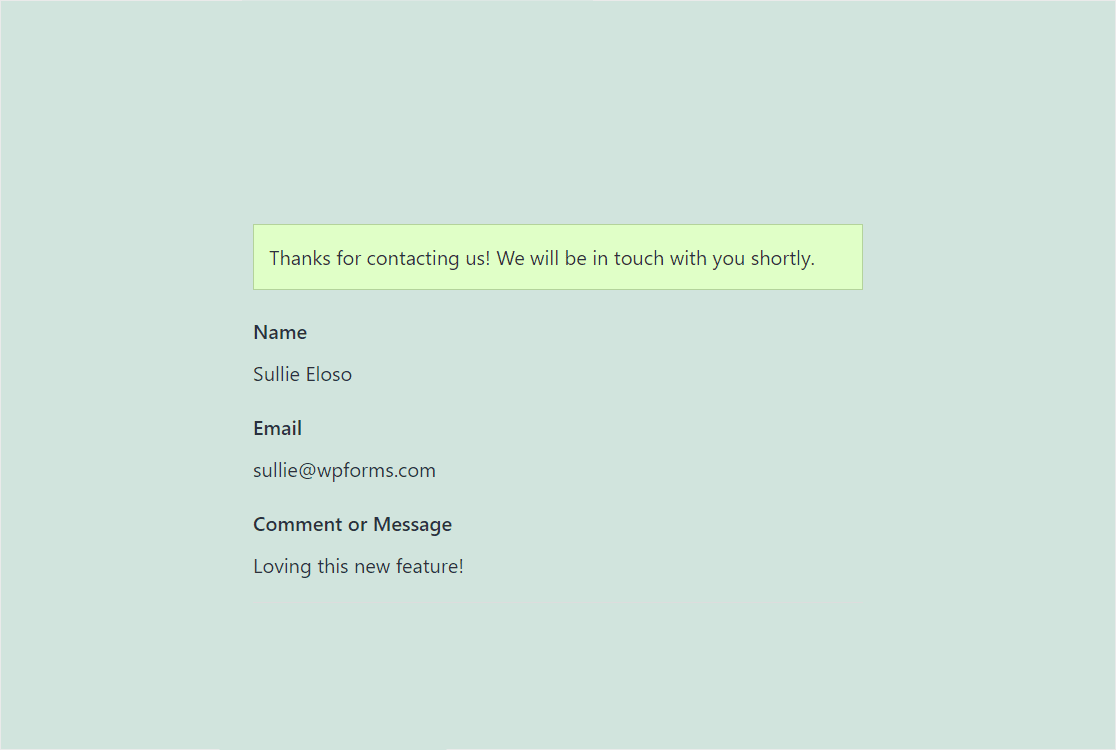The image depicts a contact page against a light green background. Dominating the top-center portion of the page is a prominent yellow box containing a message. The message reads: "Thanks for contacting us! We will be in touch with you shortly." Below this, user details are listed in a neat format: 
- **Name:** Suli Aloso
- **Email:** Suli@wpforms.com
- **Comment or Message:** Loving this new feature! 

The overall design is minimalistic, focusing on clear communication with no additional elements besides the text on the green background.